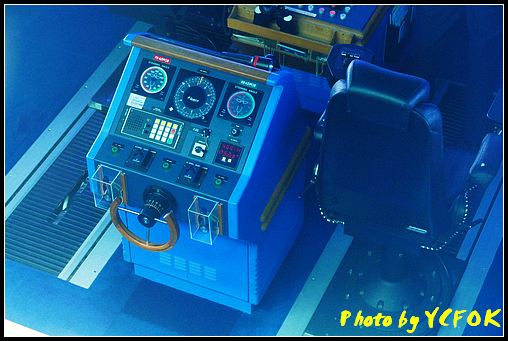This computer-rendered, overhead view depicts a detailed navigation panel aboard a seafaring vessel. At the forefront is a half-circle steering wheel, flanked by numerous digital and analog readouts. Prominently featured are three circular analog gauges in the top row, accompanied by a set of multicolored buttons beneath them. Adjacent to this main control panel is a bolted swivel captain's chair with armrests, positioned to the right. Another complex equipment panel extends in front of the primary control console. The entire image is predominantly blue with slightly blurred edges. In the lower right corner, messy bright yellow handwriting reads “photo by YCFOK.”